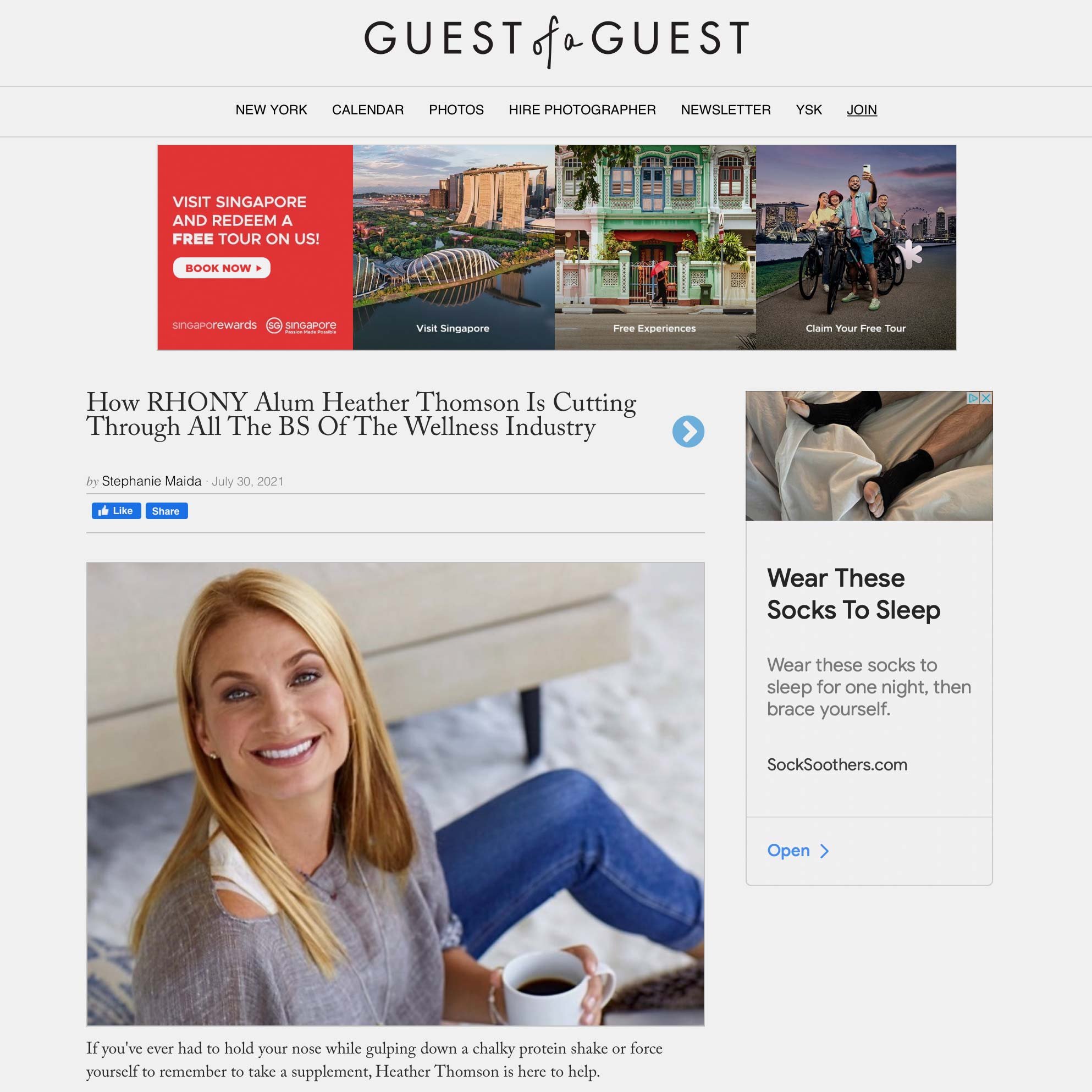The screenshot captures a webpage from the online journal, "Guest of a Guest." At the top of the webpage, there are several navigation options: New York, Calendar, Photos, Hire a Photographer, Newsletter, YSK, and Join. 

Below these options, an embedded advertisement is prominently displayed, inviting users to "Visit Singapore" and redeem a free tour by booking now. To the right of this ad, there are three images related to the promotion: the first image shows an aerial view of Singapore with the caption "Visit Singapore," the second promotes "Free Experiences," and the third encourages users to "Claim Your Free Tour."

Further down, the main article titled "How Rony Alan Heather Thompson is Cutting Through All the BS of the Wellness Industry" can be seen. A large photograph accompanying the article depicts Alan Heather Thompson, assumed to be the subject of the piece. In the image, she is holding a coffee mug and gazing into the camera. She is dressed in blue jeans and a casual linen top. The text beneath the photograph appears to be the beginning of the article.